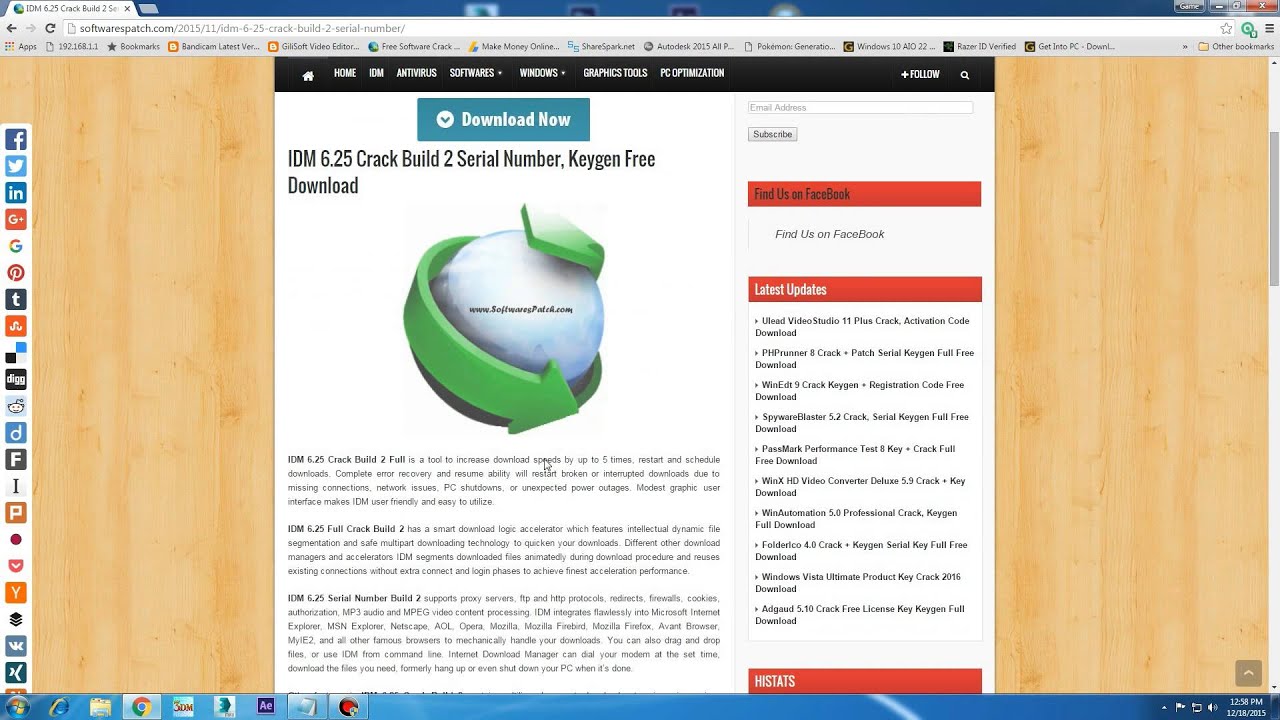The image is a screenshot of a website displayed on a computer screen. On the left side of the screen, there is a vertical toolbar featuring various app logos, including recognizable ones such as Facebook, Twitter, LinkedIn, Google+, Google, and Pinterest, among others that are less familiar. 

At the bottom of the screen, the taskbar is visible, displaying the currently open or pinned applications, along with the system time and date. At the top of the screen, the browser interface shows a single open tab and the website URL in the address bar. 

In the center, the main content area features a light brown wooden wallpaper background with a pop-up window displaying a news article. The pop-up includes a black navigation band with white text, containing options such as "Home" and possibly other menu items that are not clearly visible.